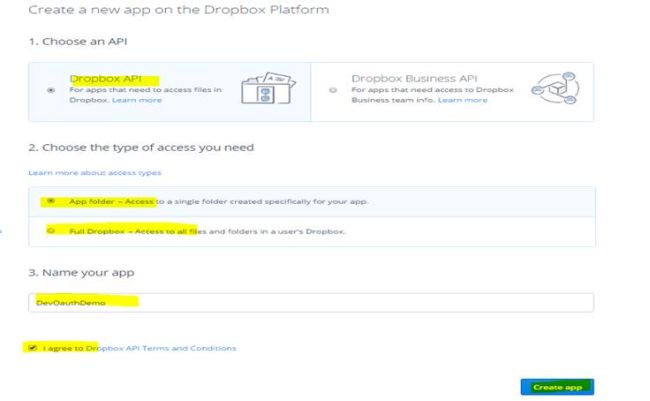The web page displayed is designed with a clean white background. At the top, in grey text, the heading reads "Create a new app on the Dropbox platform." Below this heading, the sequence begins with the numeral "1" indicating "Choose an API." This section features a horizontally split rectangular box.

On the left side of the box, with a light grey background, a bullet point marked in a circle is highlighted in yellow and designated as selected, labeled "Dropbox API." Underneath, a concise description reads, "For apps that need to access files in Dropbox," followed by a "Learn more" link and a small accompanying icon.

On the right side of the box, with a plain white background, an unselected bullet point and circle are displayed. This section is labeled "Dropbox Business API." The description here states, "For apps that need access to Dropbox Business teams info," also followed by a "Learn more" link and a matching icon.

Proceeding to the next step, marked as "2," the instruction reads, "Choose the type of access you need," with an additional "Learn more about access types" link. This section presents two text boxes. The top box is selected and highlighted yellow, labeled "App folder access," detailing that it grants access "to a single folder created specifically for your app." The second, unselected box reads, "Full Dropbox access to all files and folders in a user's Dropbox," also with yellow highlighting.

Step "3" follows, labeled "Name your app." Here, a text box is provided, already filled with the placeholder text "dev O off maybe demo," which is completely highlighted in yellow. 

Finally, there is a checkbox, which is ticked, accompanied by the text, "I agree to Dropbox API terms and conditions," with the initial part of this text highlighted in yellow.